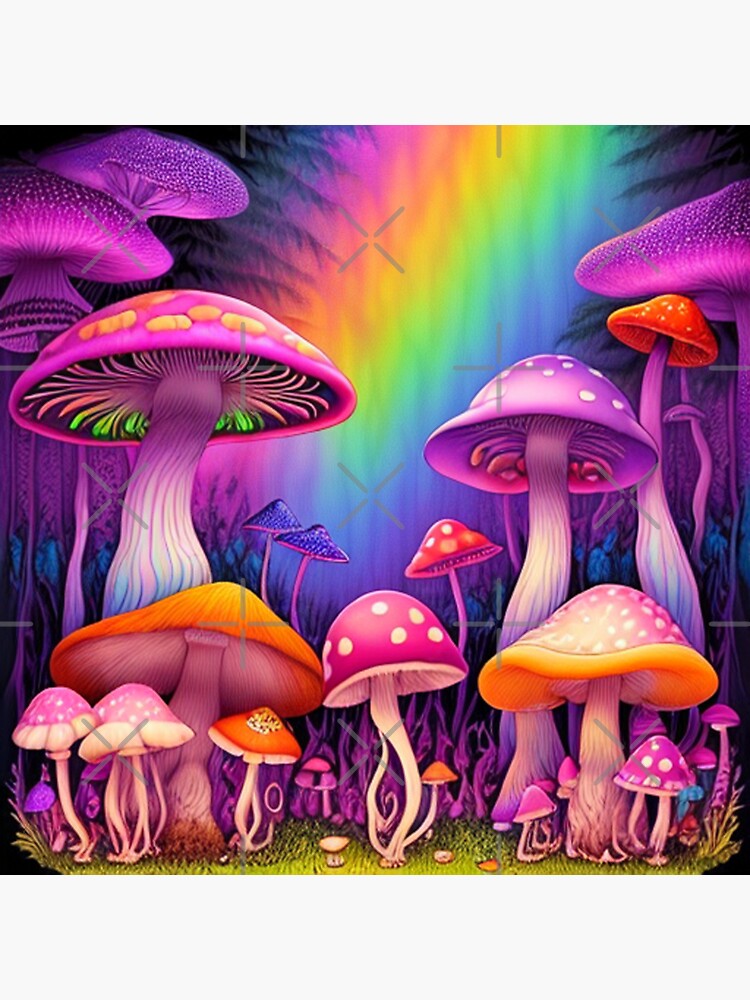This image is a vibrant, artistic rendering of an enchanting field full of colorful mushrooms, depicted in a comic or anime style. In the foreground, green grass hosts a variety of small mushrooms, some of which have little feet, giving the whimsical impression that they are walking among the others. These smaller mushrooms are predominantly pinkish with a couple of orange ones mixed in. As you move to the middle section, the mushrooms become larger, displaying a dazzling array of neon colors including pink, yellow, green, blue, red, and purple. The larger mushrooms exhibit intriguing patterns such as pink and yellow dots or pink and white dots. In the background stands a forested area, behind which a mesmerizing, rainbow-colored sky stretches out, further enhancing the magical and trippy aesthetic of the scene. The entire composition includes roughly 20 mushrooms of varying sizes and shapes, with some appearing to float in the back, their colors shifting to darker shades of pink and purple. The ground also features occasional spiky elements, adding to the overall rich texture and detail of the artwork.